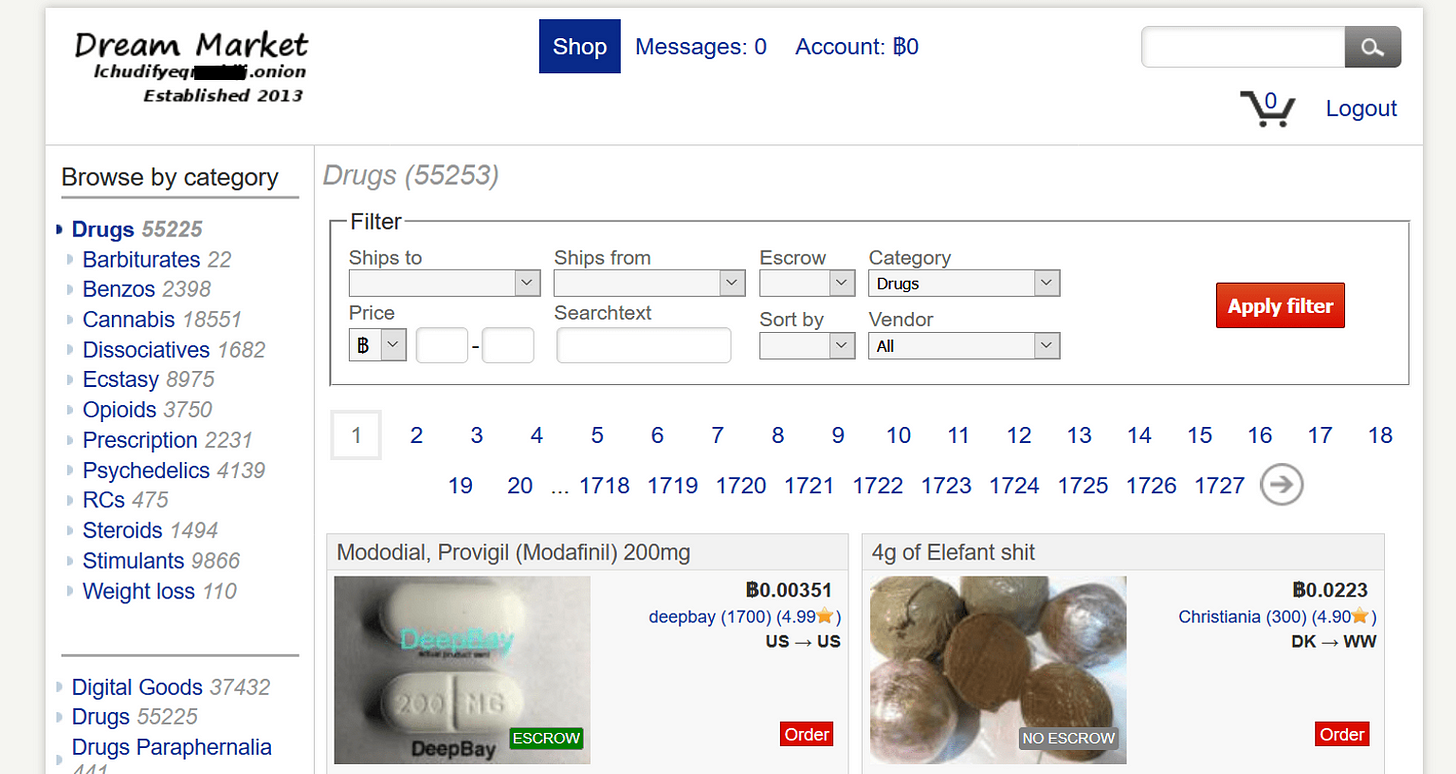Screenshot Description of Dream Market Website

The image captures a screenshot of a website named "Dream Market," which appears to be an online marketplace specializing in the sale of various drugs. The layout and design resemble typical e-commerce platforms, featuring areas for user account management, shopping, messaging, and a checkout section at the top of the page.

The website organizes its drug offerings into multiple categories: Barbiturates, Benzos (Benzodiazepines), Cannabis, Ecstasy, Opioids, Prescriptions, Psychedelics, Research Chemicals (RCs), Steroids, Stimulants, and Weight Loss products. Each category appears to have a dedicated section, likely containing listings of available substances.

A specific area on the site allows users to filter their search based on the type of drug they are seeking. Unlike conventional online stores, this website lists prices in Bitcoin, suggesting the use of cryptocurrency for transactions instead of traditional national currencies like US dollars, pointing towards an effort to maintain anonymity both for buyers and sellers.

The overall impression given by the screenshot is that of an illegal marketplace, possibly part of the darknet, where users can purchase prohibited items. The nature of the goods being sold, along with the use of Bitcoin, contributes to the perception that this is a clandestine and illicit operation.